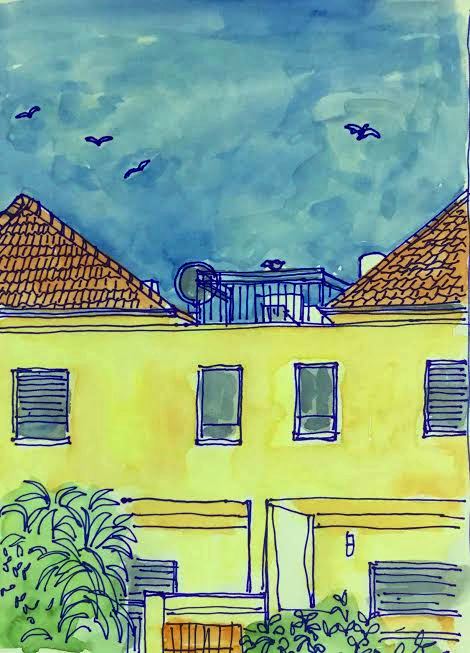This image portrays a vibrant, watercolor painting of a yellow duplex house with a distinctly cartoonish design. The house features two brown, upward-pointing triangular roofs, separated by railings and a circular object, presumably a satellite dish. The windows, outlined meticulously in a dark royal blue pen, include four on the second story—two of which have thick blue blinds. The house is surrounded by plants and shrubbery, with a bunch of green grass on the right side, painted with lines to indicate leaves. A gate is also visible in the foreground. The sky above is a rich, dark blue, created with a watercolor bleeding effect, and is populated by simple bird figures that resemble seagulls. The entire composition harmonizes the use of pen and watercolor to create a deeply intense and visually appealing scene.